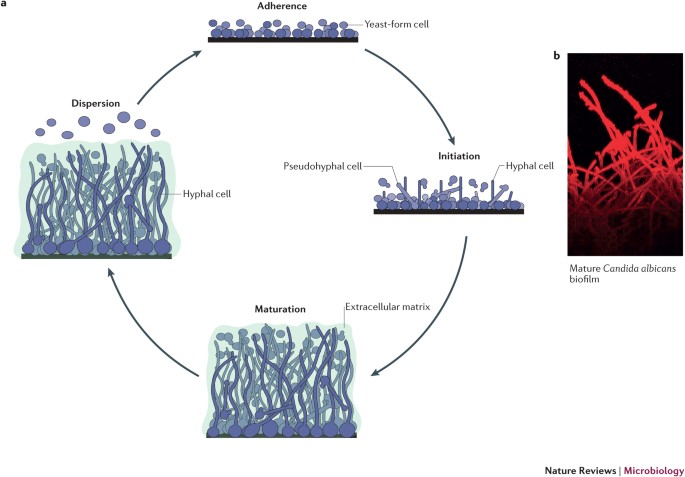The image consists of two components labeled A and B. Component A is a detailed chart illustrating the four stages of Candida albicans biofilm growth: adherence, initiation, maturation, and dispersion. The diagram is color-coded in pale green and purple, with labels for each stage. Adherence is marked by the formation of yeast cells, initiation by the growth of pseudohyphal and hyphal cells, maturation by the establishment of the extracellular matrix, and dispersion involves the release of hyphal cells. Component B contrasts sharply with the chart, displaying a close-up view of Candida albicans biofilm under ultraviolet light, depicted in red against a black background. This section highlights the dispersion stage, showing mature spores ready for distribution. The overall graphic, presented on a white base with shades of blue and black, appears to be sourced from Nature Reviews Microbiology, offering a blend of schematic and microscopic perspectives on fungal growth.